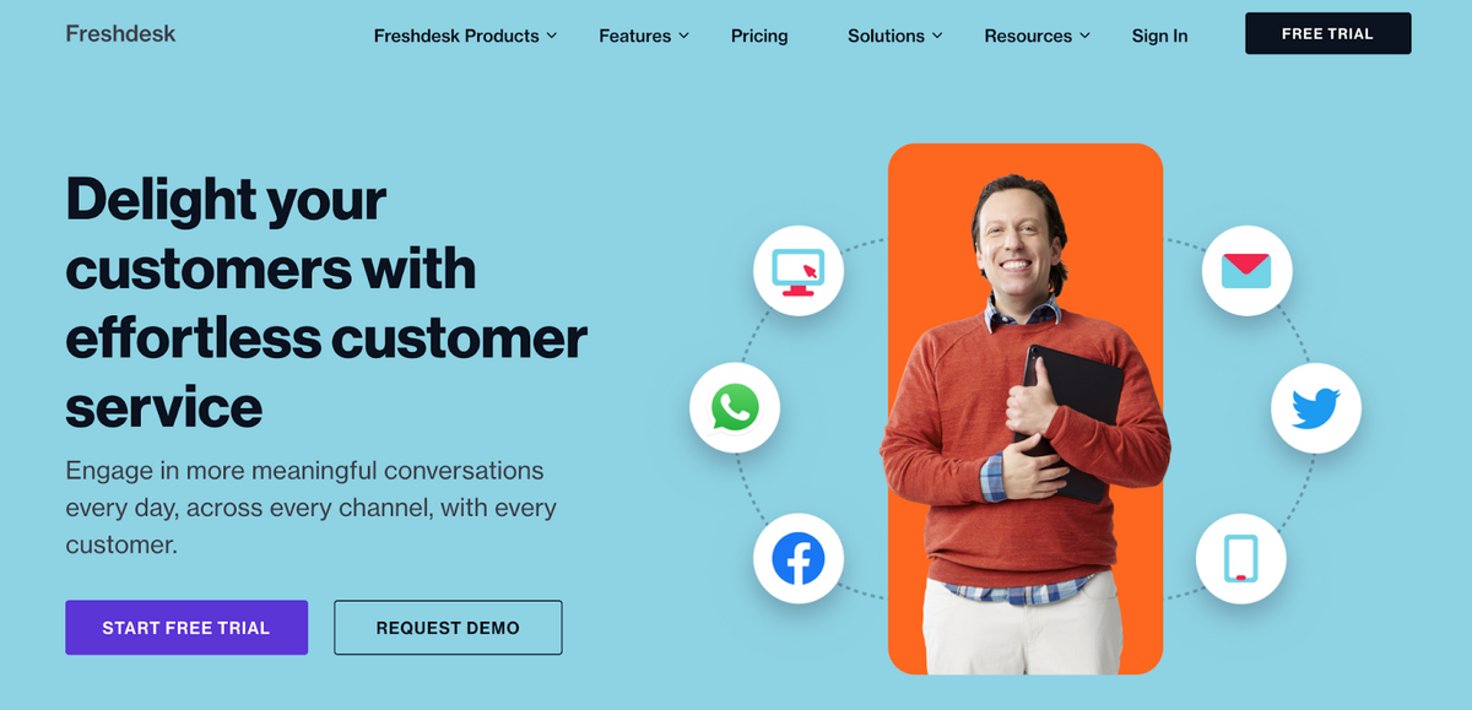This image, sourced from the Fresh Desk website, features a teal background with black text prominently displaying "Fresh Desk Products" at the top. The navigation menu includes links to "Features," "Pricing," "Solutions," "Resources," and a "Sign In" area. A conspicuous black button with white text in the upper-right corner invites users to start a free trial. Below, a headline encourages users to "Delight your customers with effortless customer service" and elaborates with, "Engage in more meaningful conversations every day across every channel with every customer."

In the lower left corner, a purple box also prompts visitors to "Start Free Trial," while a neighboring button on the right side reads "Request Demo." Central to the image is a man standing in front of an orange rectangle, holding a file folder. Surrounding him are six clickable or decorative circular icons, adding an interactive or visually engaging element to the page.